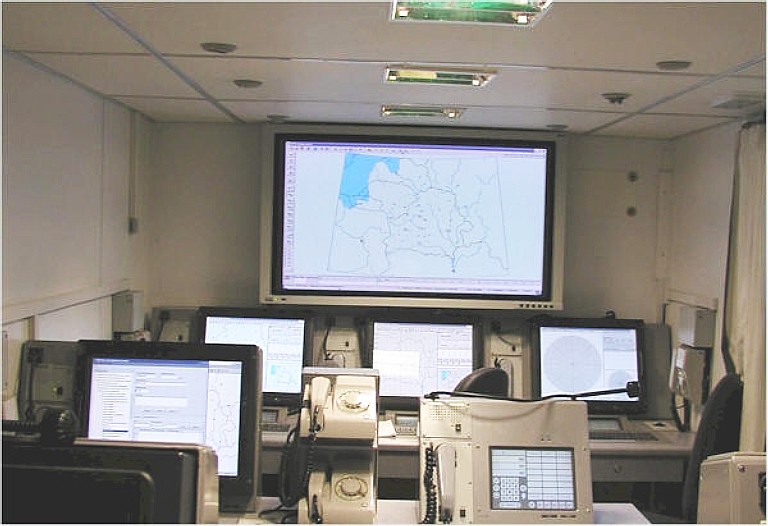This photograph, taken indoors a couple of decades ago, captures an old computer or control room setup. Centered prominently on a light gray wall is a large TV screen bordered in gray with black buttons on the lower right side, displaying a map with black and white details and a blue section in the upper left corner. Below the TV screen are three thick, black monitors placed on metal desks, equipped with older-style office chairs in front of them. Each of these monitors is paired with beige rotary phones, one on each desk. Closer to the foreground, the setup includes a black, boxy monitor displaying some indecipherable information, flanked by two older rotary phones stacked on top of each other, and another phone with an integrated screen on its right. The room features a drop ceiling with rectangular tiles, housing vents and sprinkler heads centralized, and lights aligned in pairs on either side. The overall color scheme includes white walls and ceilings, occasionally accented by the gray and beige equipment spread throughout the room. This room appears to be a station for monitoring activity, utilizing outdated technology like rotary phones and older computer systems.